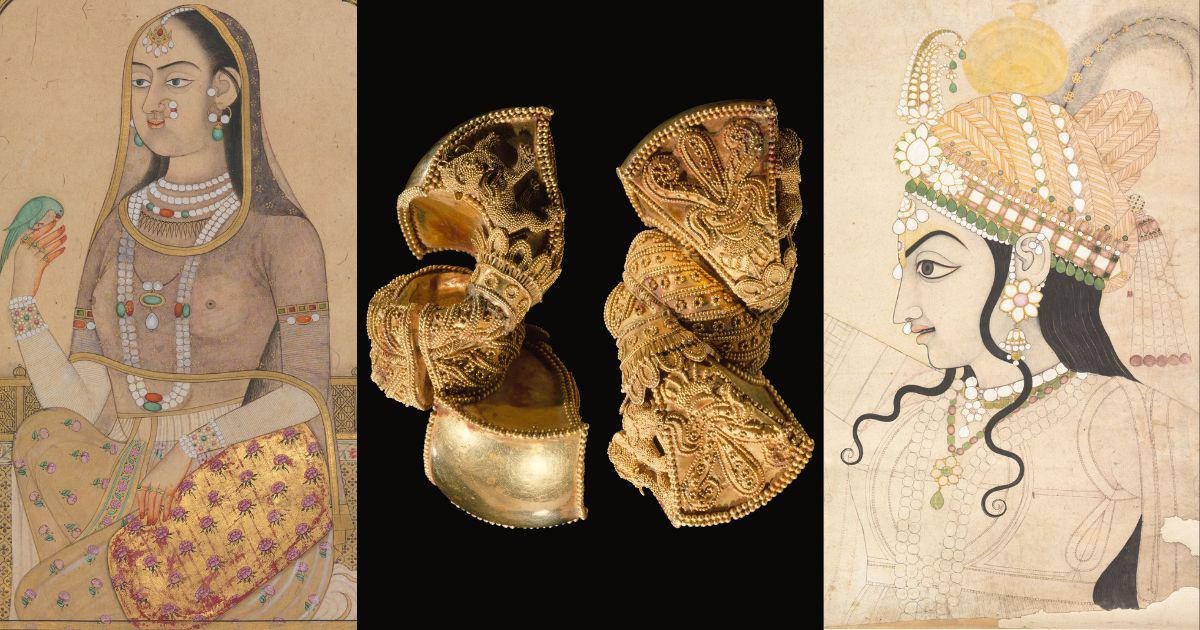The image features three panels showcasing ancient artwork and artifacts. The two outer panels depict elegant women, traditionally attired, with similarities to both Indian and Egyptian princesses. Both women are adorned with detailed garments and jewelry; one wears a sheer, see-through top while the other dons a unique headdress with curly hair and a necklace. The central panel features gold artifacts that appear to be intricate designs, possibly scarves or statues, set against a black background. A blend of cultural artistry is evident, capturing the essence of ancient opulence and craftsmanship.